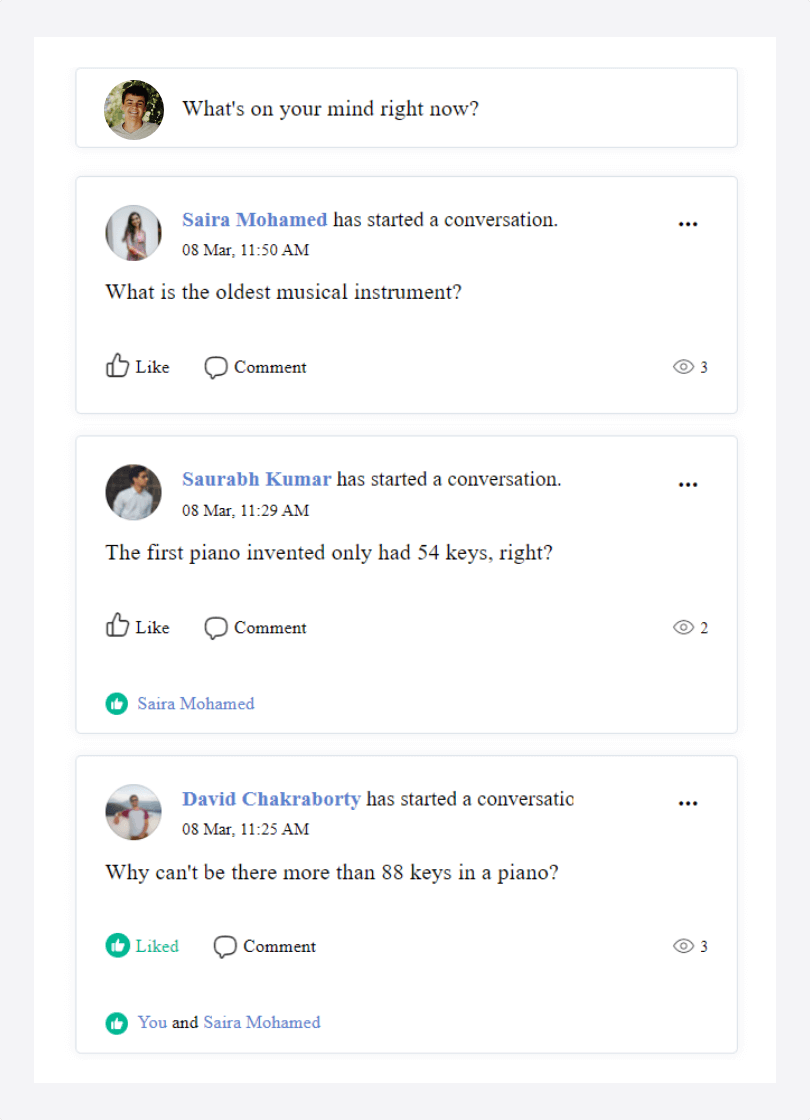This image is a screenshot of a text conversation occurring on a social media or messaging platform. The conversations are organized in small gray boxes against a white background.

At the top, there's a user interface element displaying a person's profile picture in a circle alongside the prompt "What's on your mind right now?"

Below this, the first text box features a conversation started by someone named Sarah, indicated with a date and time stamp. Sarah's question is "What is the oldest musical instrument?" This post has interactive options allowing users to like or comment on it, indicated by small icons. An icon resembling an eyeball followed by the number three implies that three people have viewed this post.

The next text box introduces a conversation initiated by a user named Saru, who asks, "The first piano, then it only had 54 keys, right?" Like the previous box, this one also includes options to like or comment. Notably, there is a green thumbs-up icon from Sarah, indicating her approval of the question.

At the bottom, another conversation box showcases a question from David, who poses another inquiry related to pianos. This post shows that it has been liked, as indicated by the green thumbs-up icon, with the added note "you and Sarah have liked this."

Overall, the image captures a series of inquisitive and interactive posts about musical instruments, with visible engagement from multiple users.